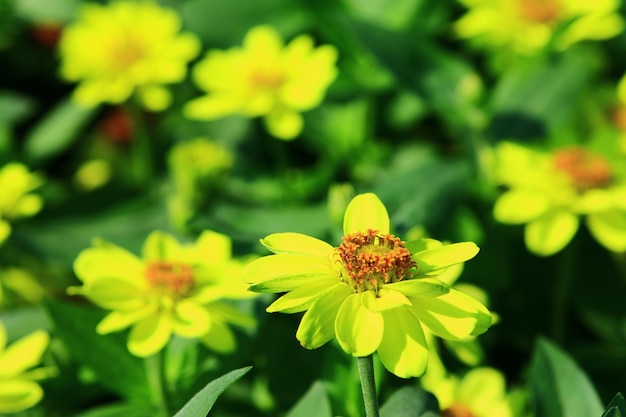This vibrant photograph captures a striking close-up of a neon green daisy-like flower with intricate details. The flower, located prominently in the lower right-hand quadrant, features a fuzzy orange ring encircling a yellow center dense with pollen. Approximately 10 to 12 silky smooth, elliptical petals, slightly concave and vividly green, radiate outward from the center, each showcasing subtle light green ribs. The flower is sharply in focus, standing out against a background of similarly vibrant flowers and teardrop-shaped leaves, all rendered in a soft blur. This effect accentuates the flower's delicate textures and bright colors, which appear almost overexposed, lending a surreal, illuminated quality to the scene. The single green stem and a finely detailed leaf add depth to this captivating botanical display.